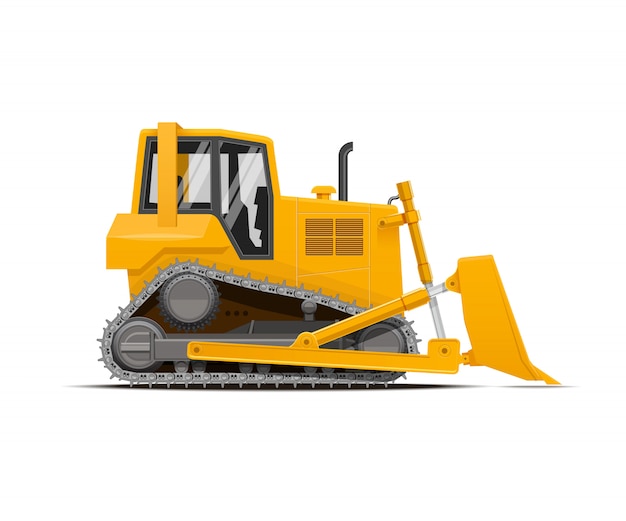The image is a detailed side view drawing of a yellow-orange caterpillar loader against a white background. The loader, captured from its right side, features a large bucket or shovel at the front with a hydraulic press behind it, indicating its ability to lift and tilt. The vehicle is equipped with tank-like tracks rather than wheels, colored in gray, and structured in a triangular shape with two round sections at the back and one at the front. The cab, framed in black, has reflective glass windows for the driver, although it is currently unoccupied. Notable details include a shining glass surface, a black stem pipe protruding from the hood, and a heat ventilation grid. The overall appearance suggests a CAD sketch of a construction vehicle designed to move and lift heavy materials.